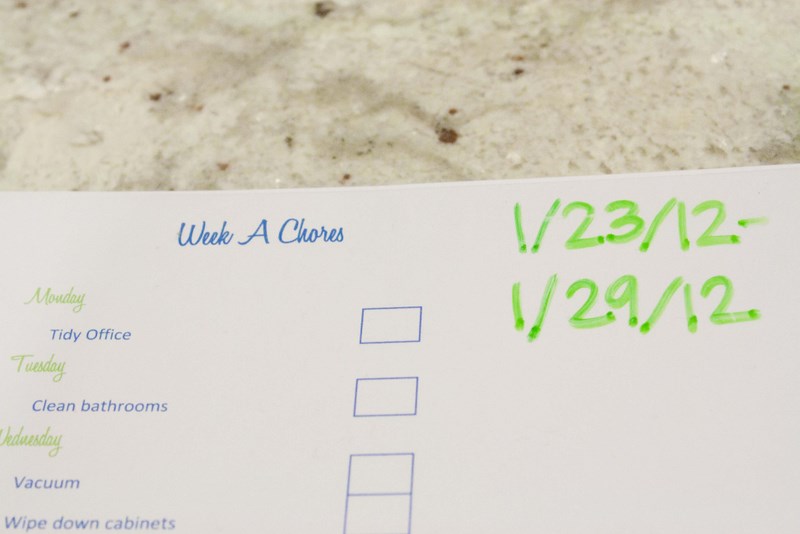The close-up photograph captures a white sheet of paper titled "Week A Chores" in elegant blue script, laying on a white marble countertop speckled with rust-colored flakes, white sparkles, and gray swirls. The top half of the image prominently features the countertop, while the bottom half showcases the chore list. The sheet is likely laminated for use with dry-erase markers. Each day of the week is color-coded in green handwriting, with corresponding chores written in blue font. For Monday, it lists "Tidy Office" with an adjacent empty checkbox. Tuesday follows with "Clean Bathrooms" and another checkbox. On Wednesday, there are two tasks: "Vacuum" and "Wipe Down Cabinets," each paired with an empty checkbox. In the upper right corner of the paper, dates "1-23-12" to "1-29-12" are handwritten in green marker, denoting the specific week for these chores.